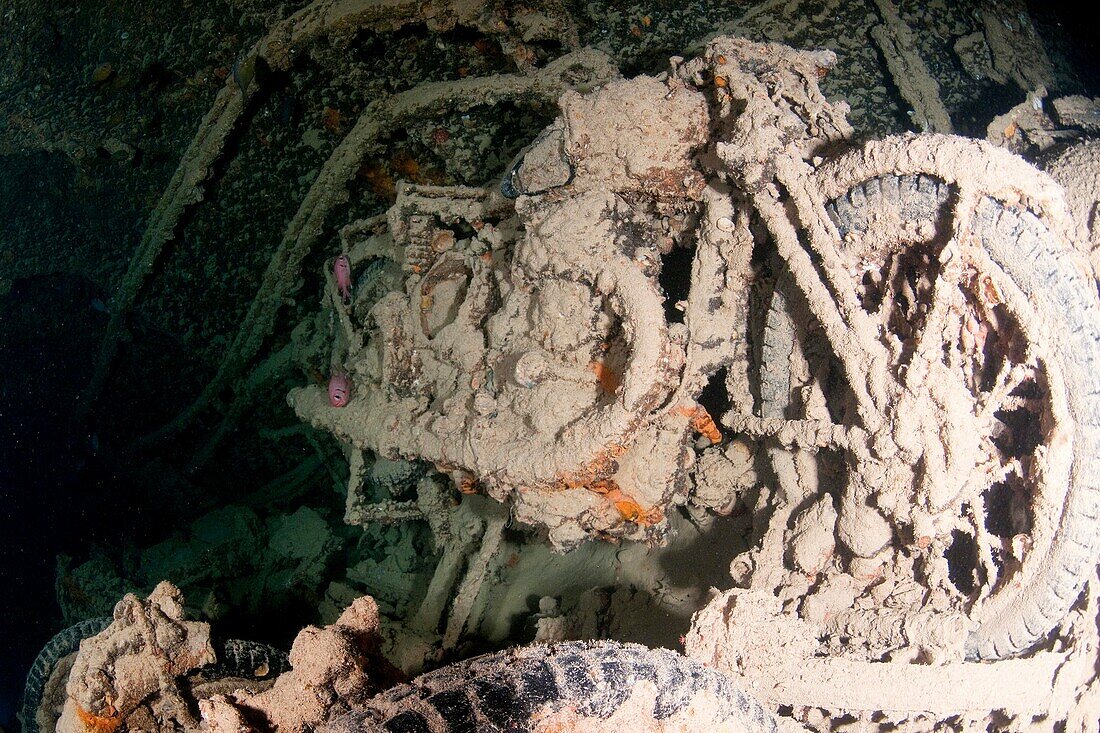This is an underwater photograph of a sunken motorcycle, heavily caked in a creamy tan sediment and various underwater growths including barnacles. The motorcycle is facing to the right, with its front wheel prominently visible and encrusted in dried mud. The engine area, visible to the left of the front tire, shares the same thick, dried mud covering. The colors in the image are predominantly shades of tan and sandy brown, with the left side of the photograph fading into darkness. Distinguishable features such as the tire spokes and parts of the engine are visible, while the rear portion of the motorcycle is obscured by shadows. Additionally, there are faint glimpses of other tires near the lower edge of the image, similarly encrusted. Small fish can be spotted swimming around, reinforcing the underwater setting. The image is devoid of any text or watermarks, and overall, the right side is brighter with pale light illuminating the motorcycle, while the left side is darker, possibly hinting at a cave-like background.